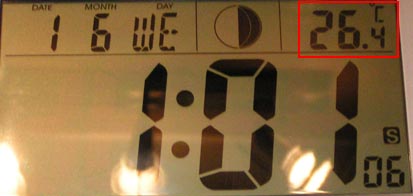The image features a gray digital screen displaying a multitude of information. At the top left, the date is shown as "1.06" for June 1st. It is followed by "Wednesday" abbreviated as "W.E.". Adjacent to this, a partially shaded circle represents a half-crescent moon phase. In the top right corner, a red square encloses the temperature "26.4°C". Dominating the lower part of the screen, large text reads "1:01 PM" with seconds "06" in smaller text beside it. Additionally, there are visible light glares across the screen, adding to the reflective quality.